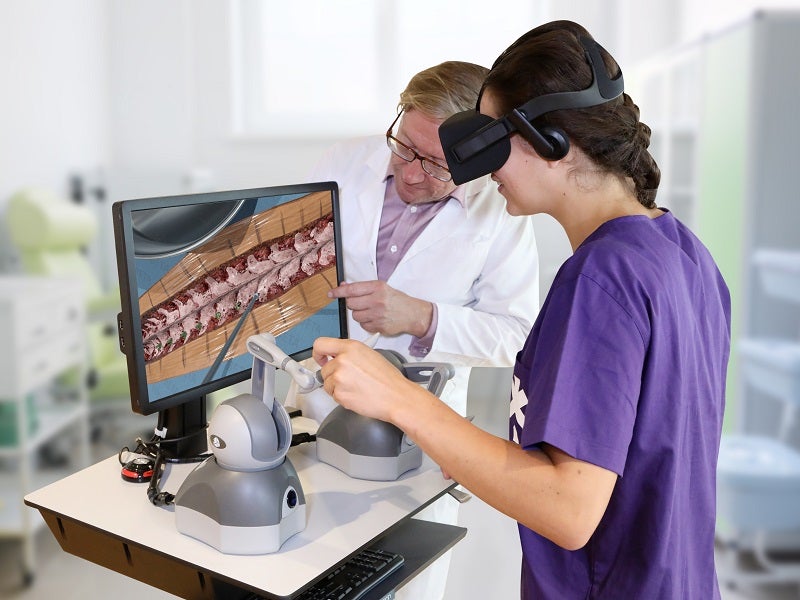In this detailed image, we see two individuals, likely in a medical or scientific setting, engrossed in a computer screen displaying an anatomical image with a teeth pattern on a blue background accented with yellow at the top and bottom. The female on the right, wearing a purple shirt, has her back turned to the camera, showcasing her black hair pulled back in a braid and virtual reality glasses perched on her head. Her hands grip two gray and white remote control devices on a white square platform, possibly for guiding a medical procedure or simulation. Beside her, to the left, stands a male figure, donned in a white lab coat with a purple undershirt visible underneath. He has blonde hair and glasses, and he is pointing intently at the lower right corner of the computer screen. The background elements are blurred, emphasizing the focus on the two individuals and the digital image they are scrutinizing.